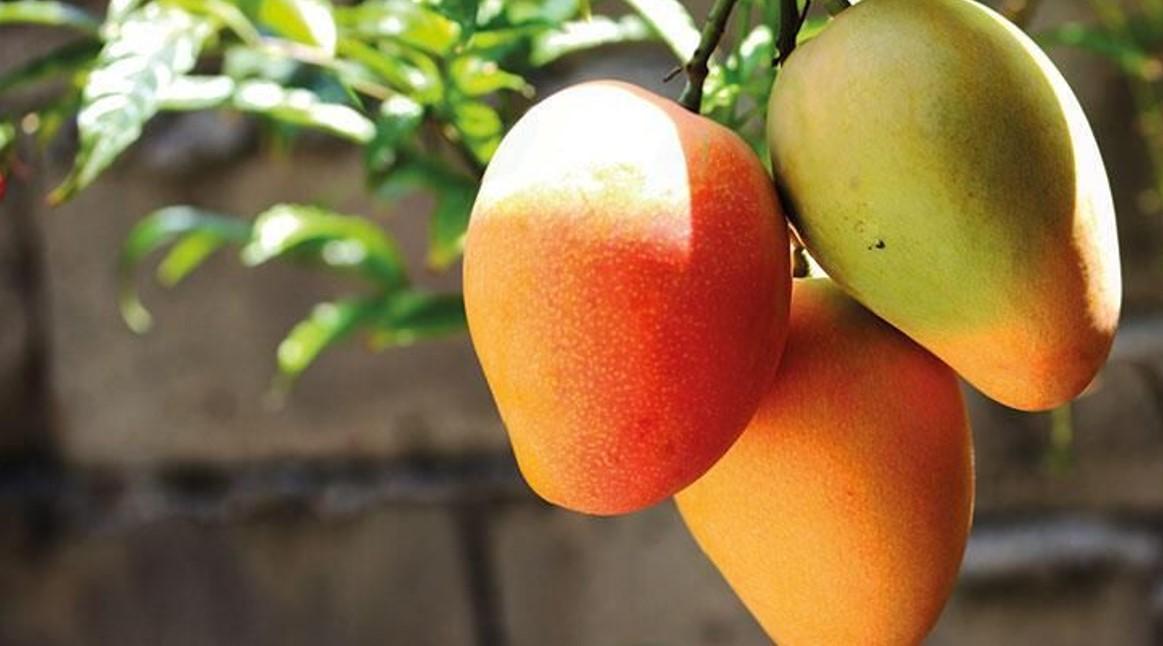In this vibrant outdoor photograph taken on a sunny day, three mangoes are clustered together, hanging from a mango tree and positioned towards the right side of the image. The mangoes exhibit a range of ripeness: the top one displays an almost ripe complexion with shades of red-orange to peach, the second is a deep orange, and the third remains largely green with a hint of orange. The fruits have an elongated, oval shape with pointed bottoms and are nestled closely, appearing to rest against one another. Direct sunlight bathes the top half of the ripest mango, casting the lower orange and green ones mainly in shadow. The background features a blurred, dark brown stone wall and softly focused leaves of the tree, capturing the essence of a sunlit day while emphasizing the vivid details of the mangoes in the foreground.